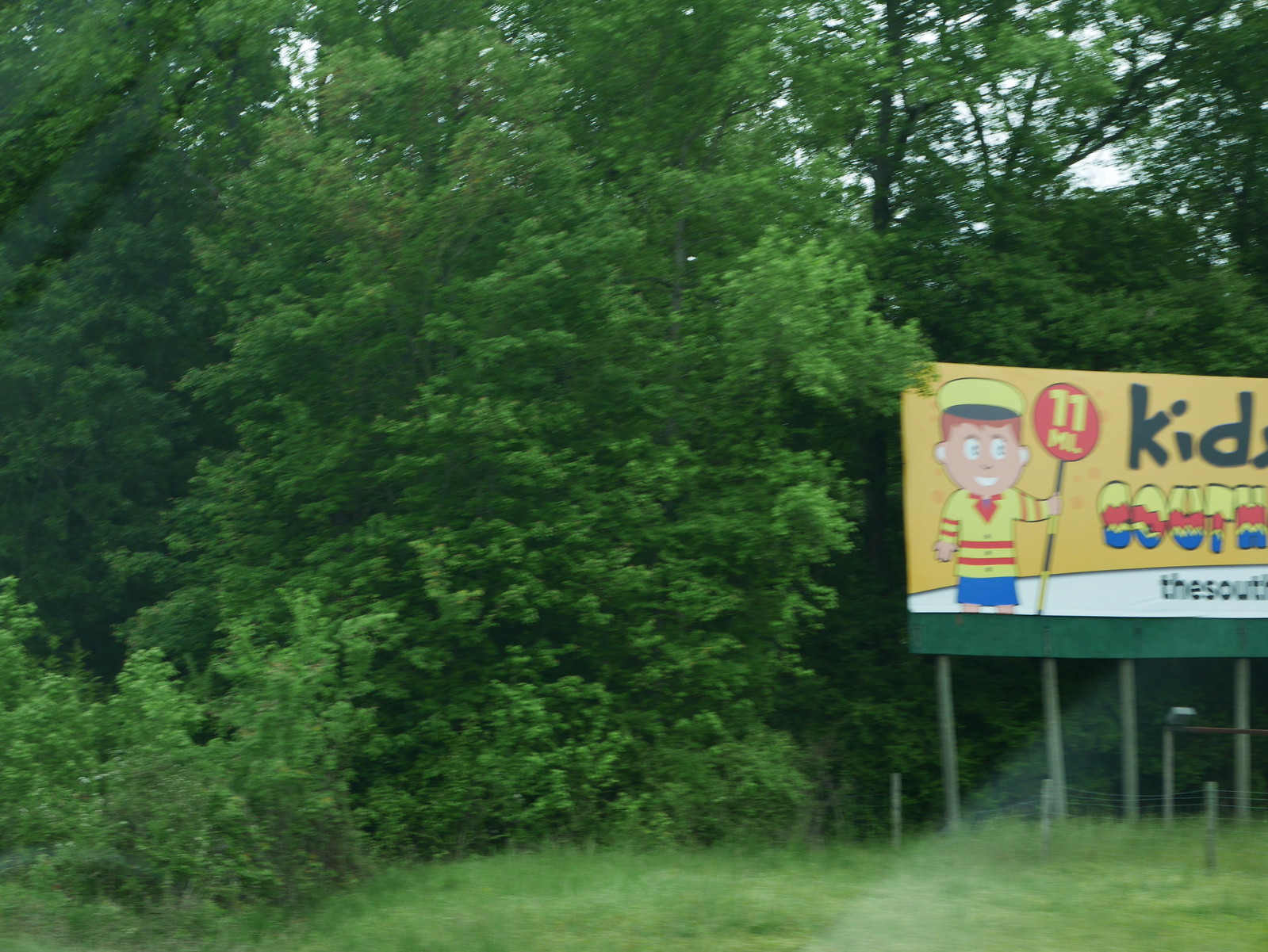This outdoor scene is enveloped in lush greenery, dominated by a vibrant canopy of green trees that occupy most of the image. A glimpse of the sky peeks through the upper background, though it is largely obscured and appears as a uniform expanse of white behind the treetops. The foreground features a lush carpet of green grass, stretching across the bottom of the image. 

On the right side, a billboard stands prominently. The left side of this billboard displays a vibrant artwork depicting a child. The child is adorned in a yellow and black hat and wears a yellow top paired with red shorts and blue shoes. The child’s left hand is raised, holding a sign, though the content of the sign is not specified in the image. The overall scene is a quaint blend of nature and human elements, highlighted by the colorful illustration on the billboard.